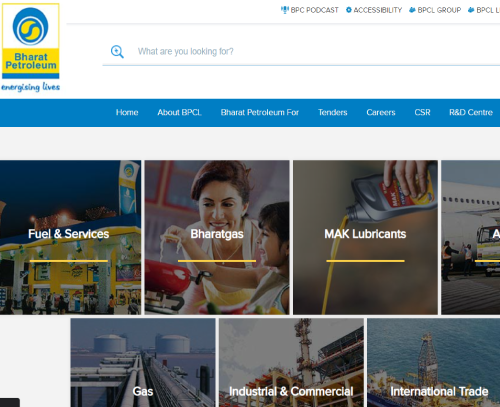The webpage for Barat Petroleum features a vibrant header in yellow and blue colors located at the top left corner, adorned with the tagline "Energizing Lives" and a small, unspecified symbol. Accompanying the header is a search bar with a magnifying glass icon, allowing users to search for content on the site. The topmost menu includes quick access links to the "BPC Podcast," "Accessibility options," "BPCL Group," and another undistinguished BPCL service.

Directly beneath this, the main navigation bar offers selections for "Home," "About BPCL," "Barat Petroleum 4," "Tenders," "Careers," "CSR," "R&D Centre," and more. Below the navigation bar, the webpage showcases a series of illustrative squares, each containing a representative image and title for different offerings:

1. **Fuel and Service** - Depicts a business setting.
2. **Barat Gas** - Illustrates a woman and a child at a stove.
3. **MAK Lubricants** - Features someone pouring oil from a bottle.
4. **Gas** - Displays a segment of a gas pipeline.
5. **Industrial and Commercial** - Shows an image resembling an industrial pipeline.
6. **International Trade** - Captures a ship navigating the sea.

Each square serves to visually guide the user to various sections and services provided by Barat Petroleum.